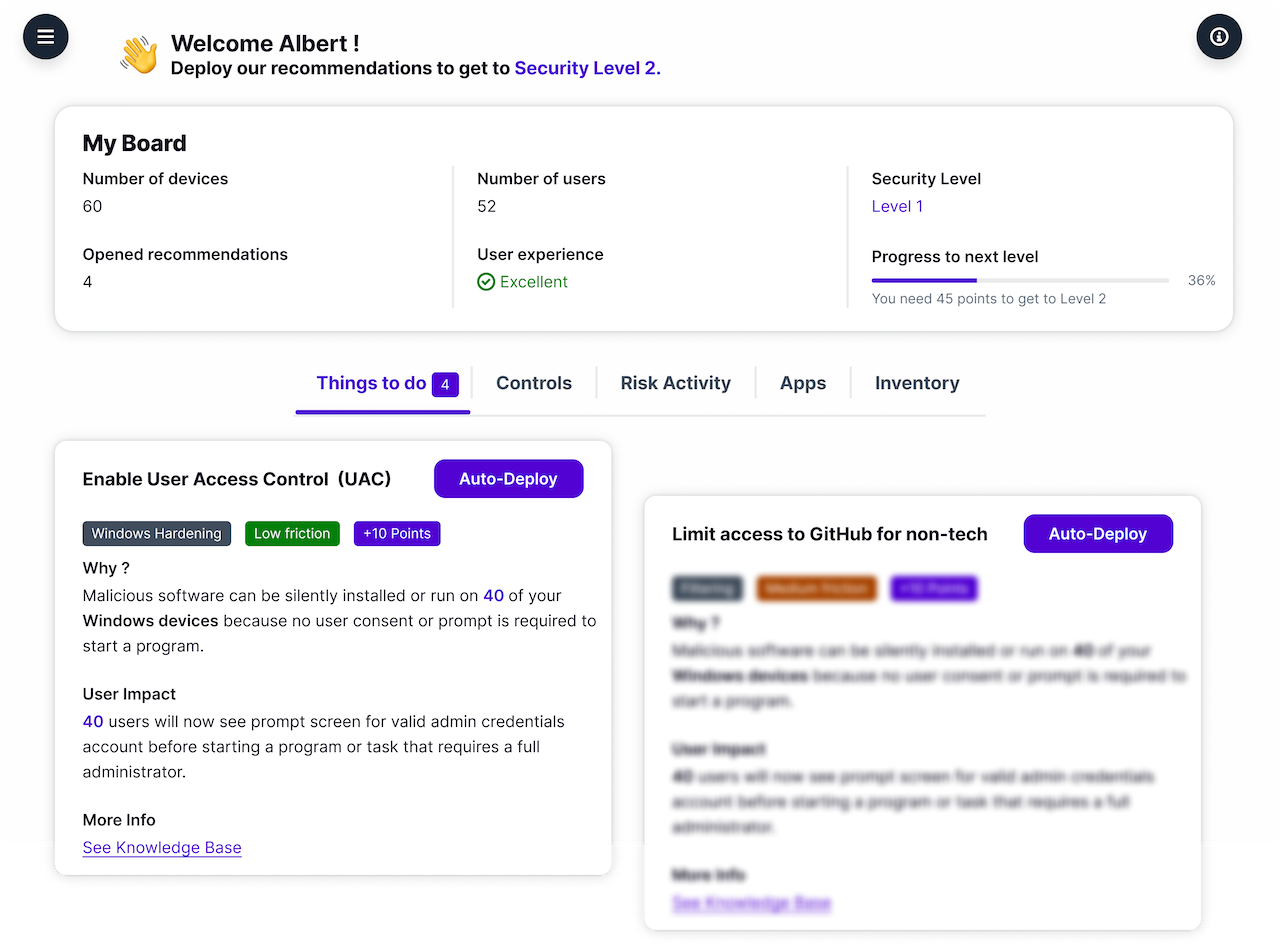This screen capture displays the interface of a computer application or website. In the top left corner, a circular button adorned with three horizontal lines indicates a drop-down menu. The upper right corner features a circular icon with an eye, suggesting the presence of additional information.

At the top of the interface, a greeting message reads: "Welcome, Albert! Deploy our recommendations to reach Security Level 2," accompanied by an icon of a waving hand. Below this, a section labeled "My Board" provides various statistics:
- Number of devices: 60
- Open recommendations: 4
- Number of users: 52
- User experience: Excellent (marked with a green checkmark).

Adjacent to these details, there is information about the current security level: "Security Level 1." A progress bar, filled to 36% with purple color, indicates progress towards the next level, noting, "You need 45 points to reach Level 2."

Further down, the interface features five tabs. The selected tab, labeled "Things to Do," has a number 4 next to it. The remaining tabs are: "Control," "Risk," "Activity," "Apps," and "Inventory."

Below the tabs are two different boxes. The box on the right has blurred out information, except for its title: "Limited access to GitHub for non-tech," accompanied by an "Auto Deploy" button. The box on the left is labeled "Enable User Control (UAC)," with an option for "Auto Deploy." It also indicates "Window Hardening," which provides a low friction enhancement worth 10 points.